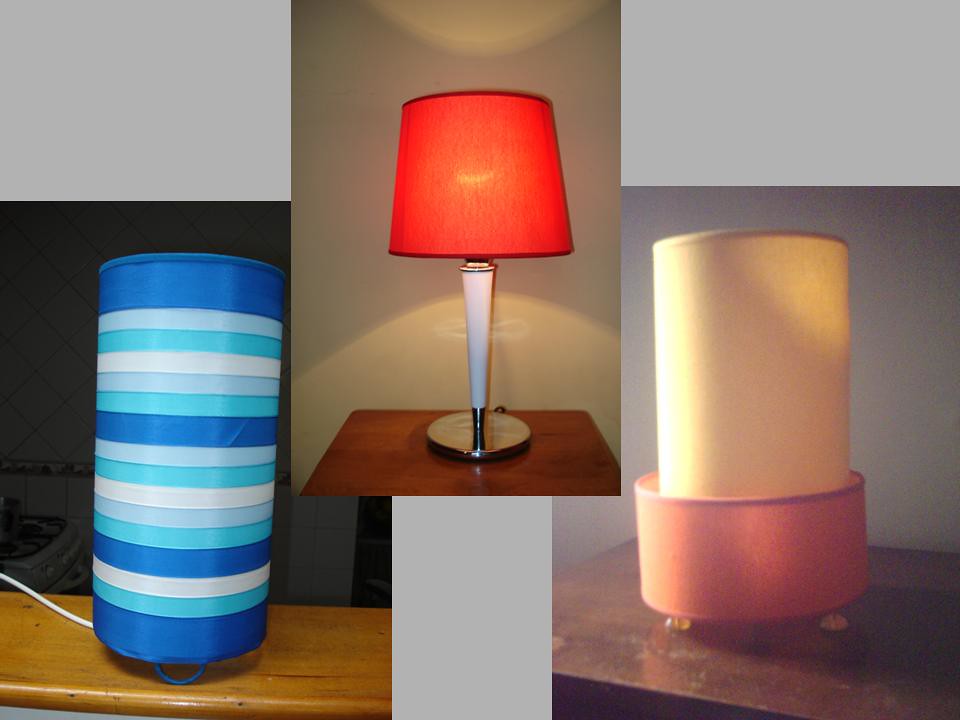This image is a composite of three distinct photographs of lamps set against a uniform gray background. The lamps are arrayed with one in the bottom left corner, another in the bottom right corner, and the third dominating the top middle, overlapping the others. 

The left lamp is cylindrical with alternating dark blue, light blue, and white stripes, reminiscent of a paper lantern fashioned from a plasticky material. This lamp rests on a wooden shelf and features a half-circle blue wire base.

The center lamp is characterized by a sleek, narrow inverted white triangle that transitions into a brass-colored base. It has an orange-brown shade that allows the light to cast a glow both above and below. It sits on a small wooden table with brass fittings visible at the top where the light bulb is housed.

The right lamp is another cylindrical structure with a white top set into a copper-colored bowl. It rests on a brown table, contributing to the varied color palette of the three lamps. 

Together, these three superimposed images create a visually engaging presentation of different lamp designs and styles, each distinct yet harmoniously arranged.